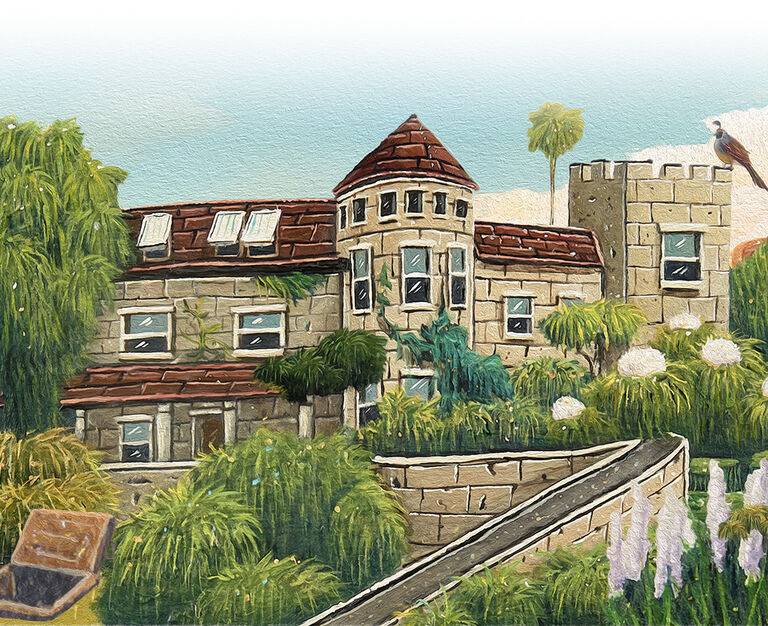This image showcases a detailed and artistic drawing of a house that bears a striking resemblance to a medieval castle. Set against a bright blue sky, indicative of a sunny day, the scene is dotted with a few fluffy clouds. The structure itself is constructed from large gray bricks reminiscent of those used in ancient castles, lending it a robust and historic appearance. The roof, made of brown wooden tiles, adds a touch of rustic charm to the castle-like house.

Near the top left of the structure, a couple of window vents protrude, hinting at a blend of traditional and modern architecture. Nearby, roughly drawn trees with long green leaves add a touch of nature to the setting. Climbing plants, possibly vines or hardy grasses, snake their way up the walls, adding to the aged yet maintained look of the building.

The façade is punctuated with roughly 10 to 15 windows, which signify a level of modernization. Among these, six small windows are aligned near the top, while a circular section of the wall features another six small windows and three larger ones, adding geometric interest and symmetry. The lower section of the building, partially obscured by the climbing plants, contains a few more windows that peek through the greenery.

Dividing the structure is a long castle wall, or possibly a moat, that extends from the middle section downwards, evoking a sense of fortification and defense. On the bottom left, there appears to be a hatch or concealed doorway, suggesting a secret entrance that harks back to the building's storied past.

Overall, this drawing beautifully merges elements of a traditional medieval castle with signs of modern habitation, set against a vibrant, sunny backdrop.